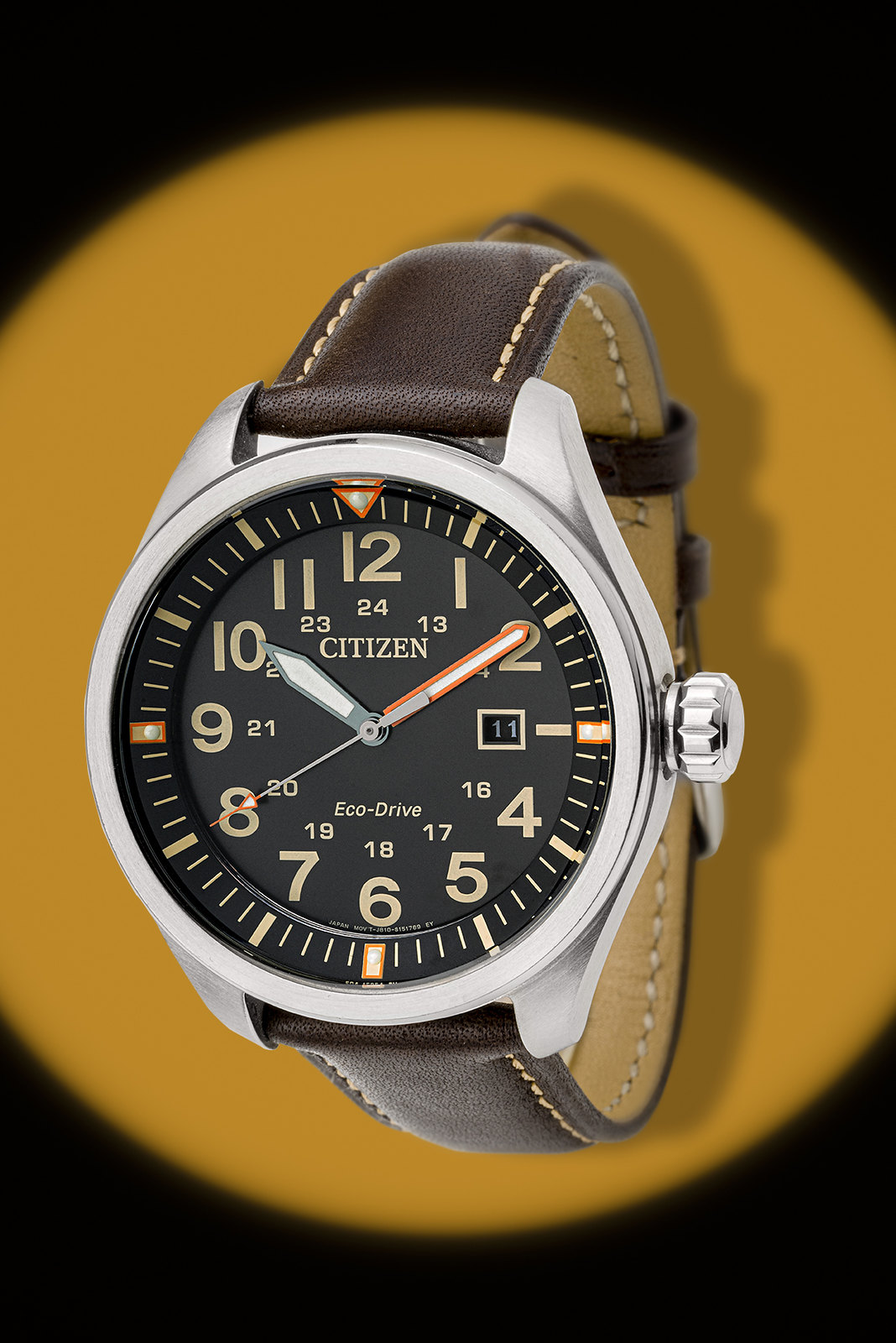The image presents a close-up of a Citizen wristwatch, captured against a dual-toned background featuring a black rectangle and an orange circle. The watch itself is positioned centrally within the orange circle, creating a striking contrast. The watch features a dark brown leather wristband with light brown coloring on the inside, and visible stitching running along the sides. Partially hidden by the watch face, the wristband is secured with a closed silver buckle. The watch face is encased in silver with a prominent, grooved silver knob on the right side. The face displays gold numerals and tick marks on a black background, with the hour hand in green and the minute hand in orange. The documented time on the watch is set to 10:10, showcasing its elegant design. The image likely serves as an advertisement or product listing, emphasizing the watch's detailed craftsmanship and aesthetic appeal.